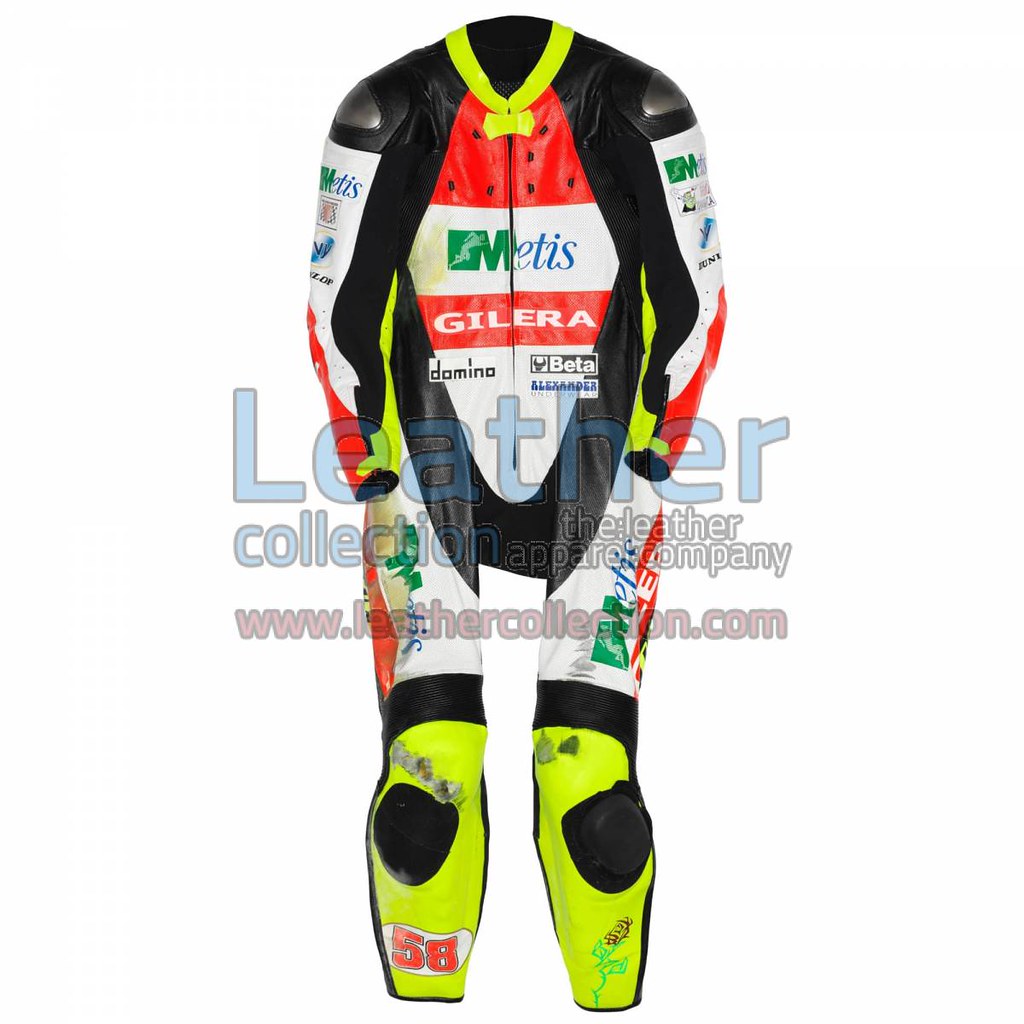The image displays a detailed motocross full-body jumpsuit set against a seamless white background. The jumpsuit is primarily black with striking highlighter yellow accents on the collar, forearms, and calves. Notably, the knees are also padded with black patches. The jumpsuit is adorned with several logos and patches, including a green 'M' and blue 'ETIS' across the chest area, followed by 'Galera' in white letters. Additional patches include a black box with 'BETA Alexander' in blue on the left side and 'Damina' on the right. The right leg features a red '58' within a white box, while a green design is present on the left lower leg. The sleeves transition from white to red towards the wrists. The image is watermarked with "Leather Collection" in blue block letters, "The Leather Apparel Company" in white, and "www.leathercollection.com" in bold red text, indicating that the product is part of a leather apparel collection, likely showcased for sale or as part of a collection display.